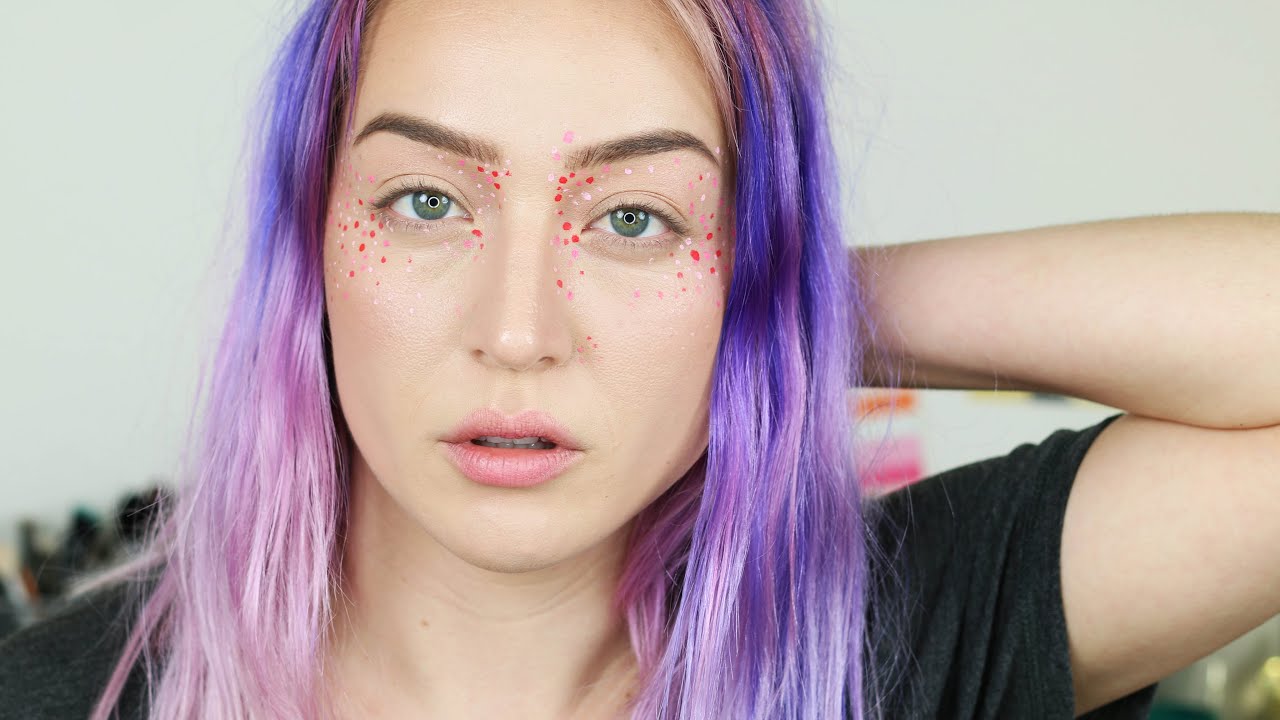The photograph is a detailed, close-up studio shot of a woman taking up approximately 85% of the frame against a plain white background. She has long, iridescent hair dyed in shades of purple, pink, and blue that transitions into lighter colors toward the ends. Her greenish-blue eyes are framed by perfectly groomed, arched eyebrows, and her light pink lips add a soft touch to her face. The woman's pale skin is adorned with intricate makeup consisting of red, pink, and white dots around her eyes, extending to the creases of her nose and slightly below it. She is wearing a black short-sleeved shirt, visible at her right shoulder and left elbow, with her left arm reaching behind her head. The overall composition and her poised look at the camera, with studio lights reflecting in her pupils, suggest a professional and artistic setting.